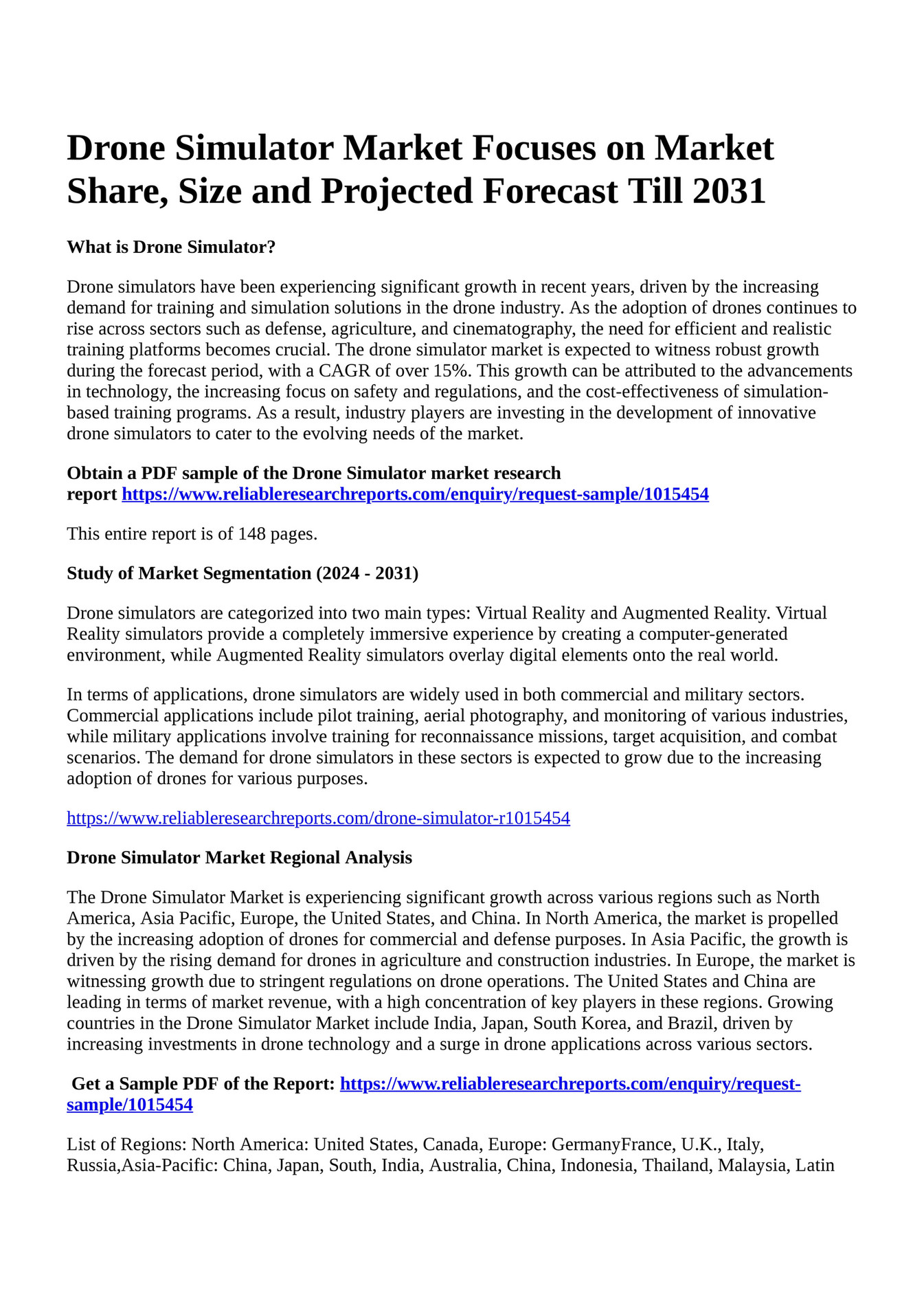The image depicts a digital document titled "Drone Simulator Market Focuses on Market Share, Size, and Projected Forecasts till 2031." The content is text-based, featuring no imagery. The document is structured into three main sections, prefaced by various headings and links to obtain a PDF sample of the comprehensive 148-page report. The first section begins with the question, "What is a Drone Simulator?" and elaborates on the increasing demand for drone simulators driven by sectors such as defense, agriculture, and cinematography, emphasizing the crucial need for realistic training platforms. It highlights a robust market growth projected at a CAGR of over 15%, fueled by technological advancements, increased focus on safety regulations, and cost-effective training solutions. The second section delves into the market segmentation from 2024 to 2031, classifying drone simulators into virtual reality (VR) and augmented reality (AR) types and listing their applications in commercial and military contexts. VR simulators provide immersive computer-generated environments while AR simulators overlay digital elements onto the real world. The final section covers the drone simulator market's regional analysis, noting significant growth across North America, Europe, Asia Pacific, and leading countries such as the United States and China. The document concludes with a "List of Regions," enumerating specific countries within North America, Europe, Asia Pacific, and Latin America.